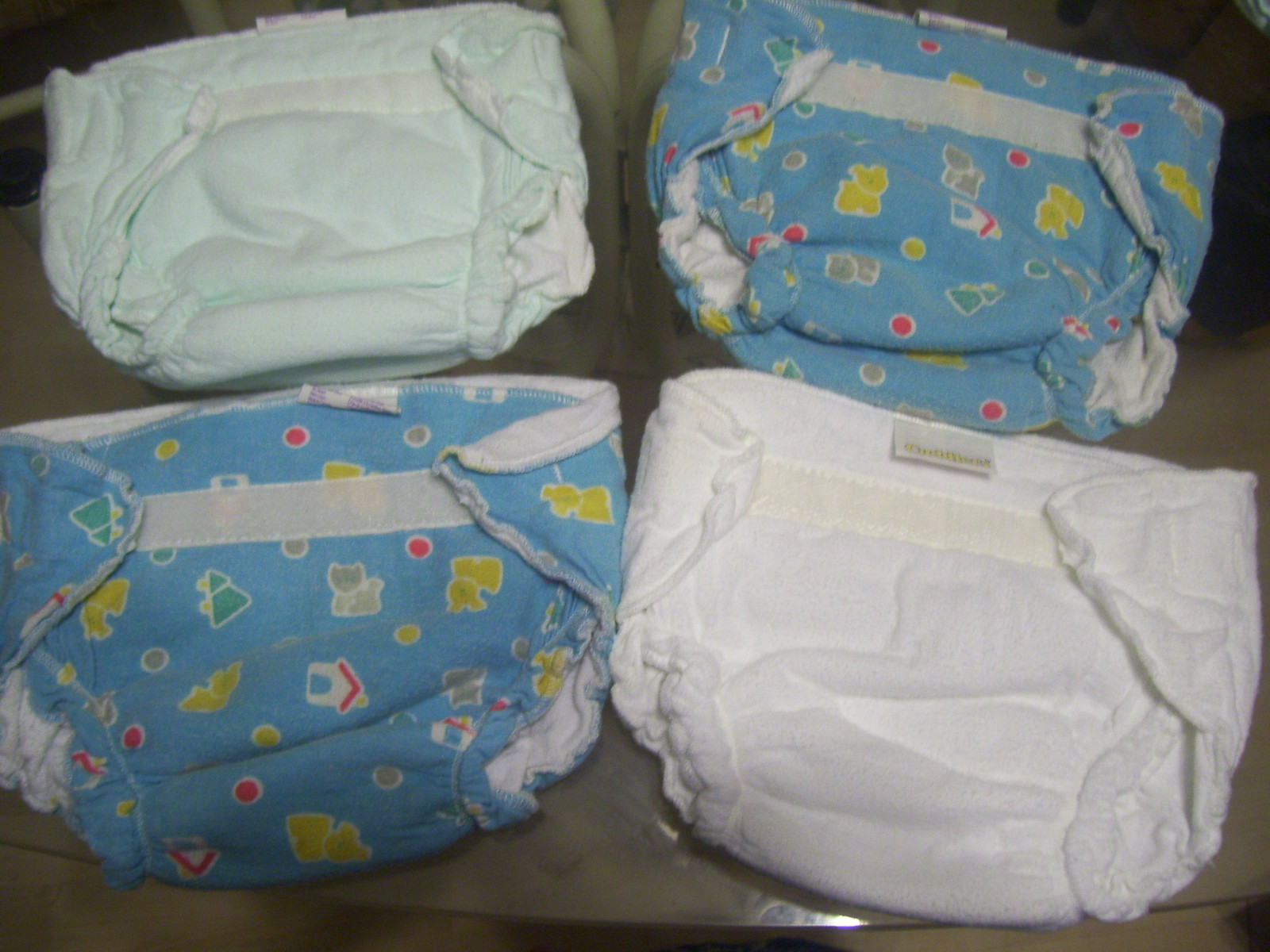This photograph captures four plush cloth baby diapers arranged in a 2x2 grid on a clear glass table. The table's background is somewhat indistinct, possibly showing white chairs or other items. Each diaper showcases unique colors and patterns. The bottom right diaper is solid white. The top right and bottom left diapers feature a medium blue fabric adorned with playful, cartoony designs, including yellow dogs, a gray cat, and red and pink polka dots. The top left diaper is a pastel mint green with a white lining, contributing to the soft, baby-themed aesthetic of the scene. The overall impression is one of variety and comfort, with a mix of solid colors and whimsical patterns suitable for a baby.